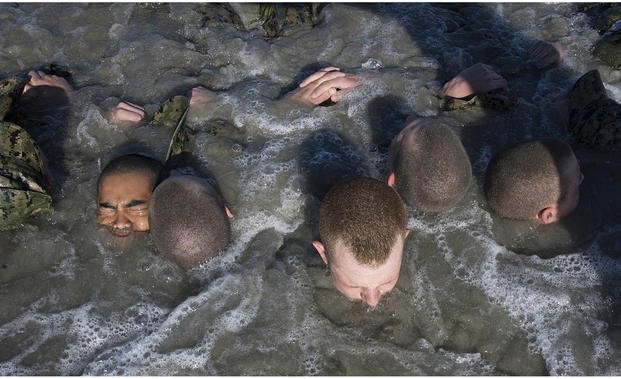This overhead photograph captures five soldiers engaged in rigorous military training, immersed in dark, foamy water, resembling a scenario akin to SEAL Team 6 exercises. The soldiers, varying in skin tones from dark to light, sport uniformly short military haircuts. Positioned close together in a circular formation, they appear to be navigating the harsh conditions, possibly struggling to stay afloat as waves crash over them.

In the image, only the tops of their heads, parts of their faces, and a few hands are visible above the waterline. One soldier on the far left has his mouth completely submerged, with only his nose, eyes, and the top of his head exposed, mud obscuring much of his face. Another, with a red shaved head, has his eyes closed and seems to be exhaling forcefully. The men are lying in opposite directions with some showing just partial faces, and their hands either on their backs or crossed over their chests, adding to the sense of a strenuous, immobilizing exercise. The scene is accentuated by a faint glimpse of camouflage in a corner, reinforcing their soldier identities in this demanding training scenario.